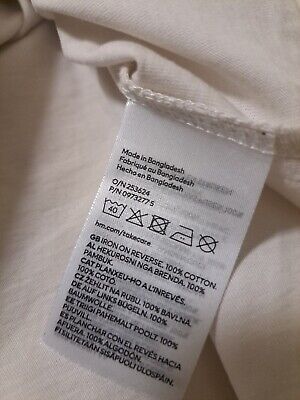The image features a standard care tag attached to a beige sheet or pillowcase. The white tag, bearing black text, specifies that the item is made in Bangladesh from 100% cotton. Prominently, the tag includes various care instructions and corresponding symbols: wash at 40°C, do not bleach (denoted by a crossed-out triangle), do not tumble dry (indicated by a crossed-out circle), and iron on reverse (signified by a simple iron symbol). Notably, it also includes the explicit instruction to use fabric softener but avoid detergent, an unusual and somewhat confusing directive. The tag's washing and care information is presented in multiple languages, including Spanish and German, to cater to an international audience.